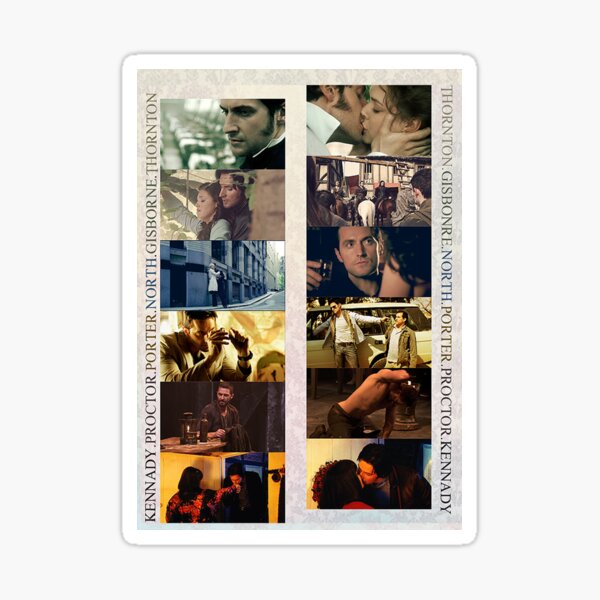A multi-paneled collage of movie scenes captures an array of dramatic moments. In the top left, a close-up of a man's face reveals an intense, brooding expression. To his right, a passionate kiss between a man and a woman exudes deep emotion. Below and to the left, another scene shows a man holding a woman in an embrace filled with urgency. Adjacent to this, several men on horseback are ominously positioned under a log with ropes around their necks, suggesting a harrowing fate.

In the middle right section, a woman stands resolutely in front of a building, her posture and expression firm. Further down, a man stares seriously off-camera while holding a small glass, likely filled with an alcoholic beverage, conveying a moment of contemplation or decision. Opposite him, another man makes a hand gesture across a table, engaging with an unseen counterpart, adding to the scene's intensity.

The entire composition is set against a cream-colored, marble-patterned background, framed by a white border that gives the collage a playing card-like appearance. Along the side, names such as Kennedy, Proctor, Porter, North, Gillsborn, and Thornton are repeated, adding a mysterious or thematic hint to the arrangement. Each image within this sophisticated montage exudes drama, creating a rich tapestry of cinematic storytelling.